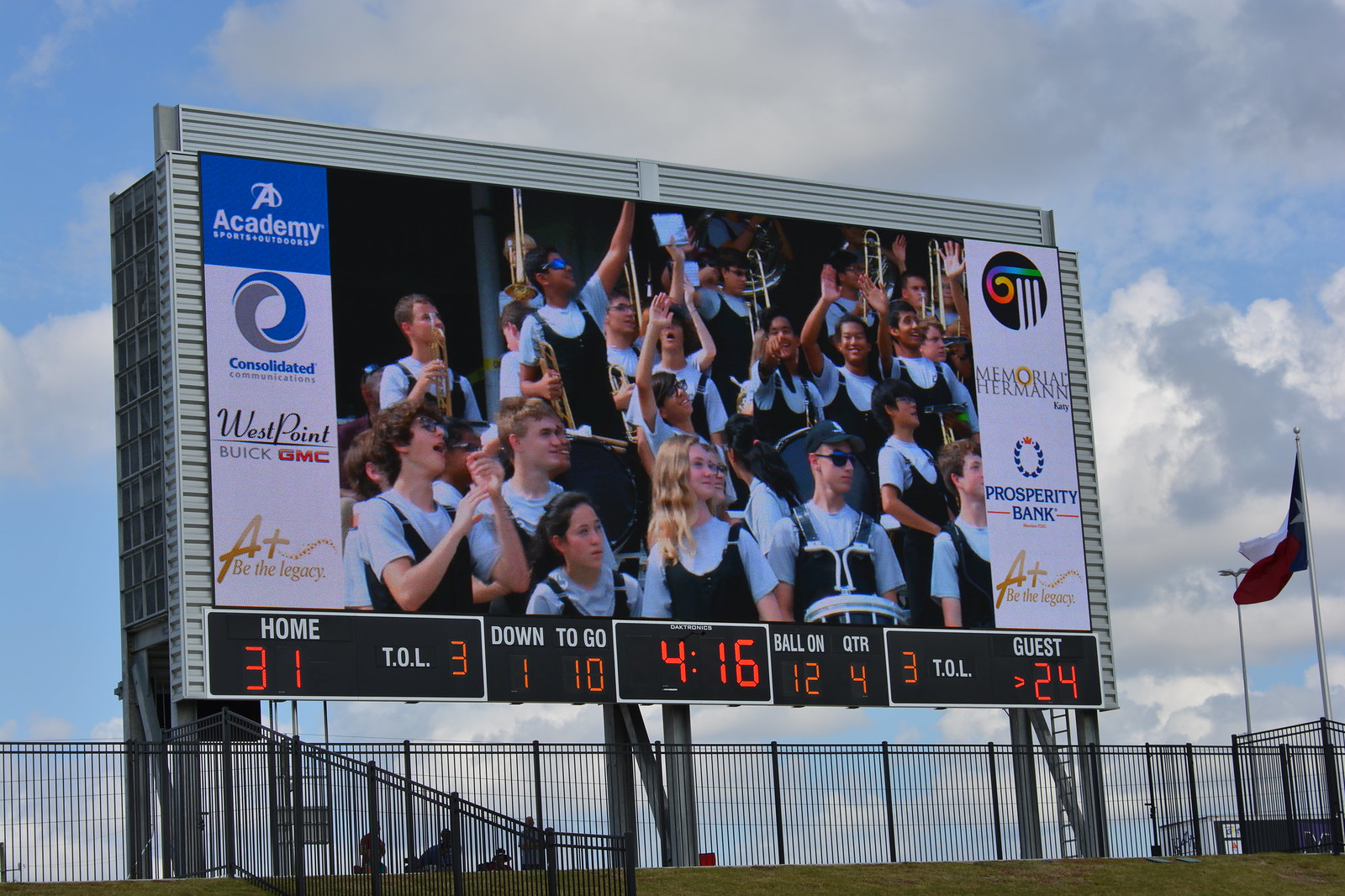This image captures a vivid, bustling scene centered around a large digital scoreboard set against a predominantly blue sky dotted with white and gray clouds. The scoreboard, taking up the middle of the photograph, features a live video feed of enthusiastic marching band students clad in black overalls and light blue undershirts, holding various instruments like drums and trumpets, joyfully engaging with the camera. The scoreboard itself displays detailed game information: "Home 31, Guest 24," with 4 minutes and 16 seconds left in the 4th quarter, and a status indicating "First Down and 10 to go," with the ball positioned on the 12-yard line. Both teams have three timeouts left. Advertisements such as "West Point, Buick GMC" border the screen on both sides. Below the scoreboard, a black fence aligns the bottom, separating it from the grassy field in the forefront. A Texas flag can be seen towards the right side of the frame, adding a regional touch. The entire setup is bathed in daylight, signifying an outdoor sports event in progress.